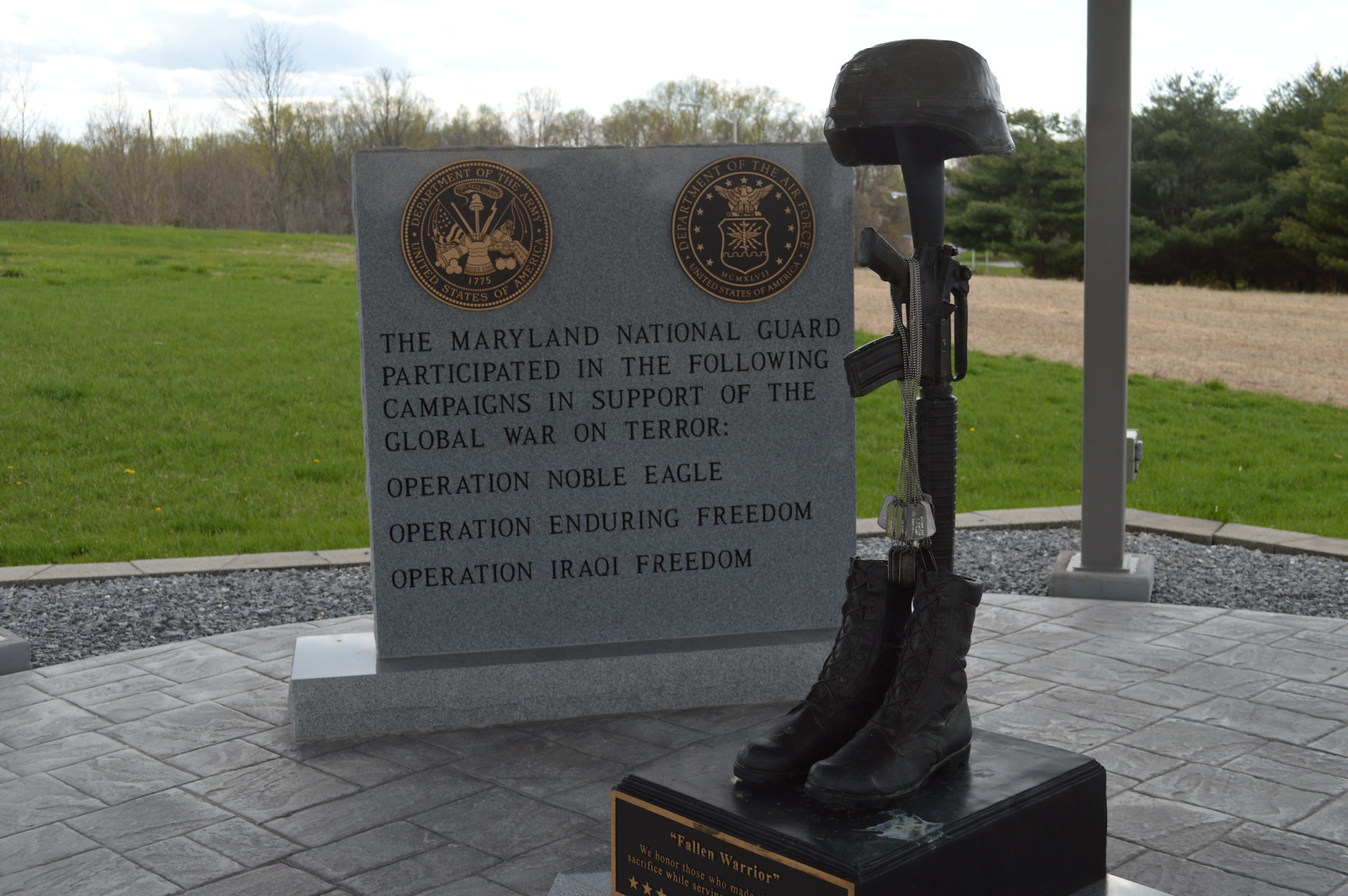This photograph captures a solemn war memorial site dedicated to the soldiers of the Maryland National Guard who participated in the Global War on Terror. Central to the image is a polished granite slab, standing tall in a small courtyard. At the top of the granite marker are two brass military seals, followed by text commemorating the Maryland National Guard’s involvement in Operation Noble Eagle, Operation Enduring Freedom, and Operation Iraqi Freedom. 

In the foreground, closer to the camera, stands a poignant sculpture depicting military boots with a rifle inverted between them, the muzzle pointing downward, and a helmet balanced atop the rifle. Beyond the memorial, the serene landscape features a lush grassy field bordered by a dense wall of trees, adding to the reflective atmosphere of the site.